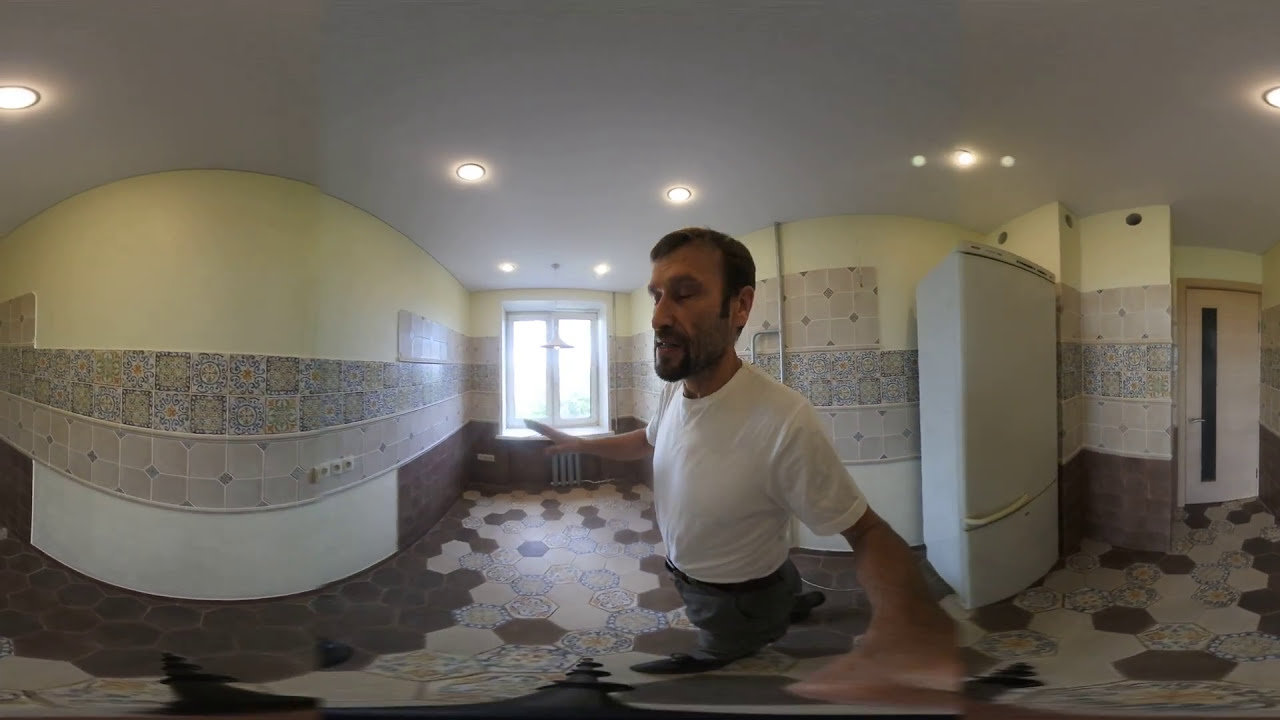This detailed color photograph, presented in a landscape orientation, is actually a composite panoramic image of a man inside a building, combining three different vantage points. The central figure is a tall Caucasian male in his mid-40s to late 50s. He has short brown hair and brown facial hair, including a light beard, mustache, and goatee. He is wearing a white short-sleeved t-shirt and gray pants. His eyes are closed, his mouth is slightly open, and he stands turned sideways towards the viewer. His left hand is holding a camera, while his right arm is extended outward. His body language is open and expressive. The background reveals a cream or light yellow interior space, possibly a public area like a lobby or a theater. The walls feature a decorative band of multicolored tiles midway between the ceiling and the floor, exhibiting patterns reminiscent of Greek, Italian, or Roman styles, with varying textures in shades of brown and gray. The floor comprises beige tiles with brown, blue, and yellow insets. To the far right, there is a tall white refrigerator. A double-sided window indicates daylight streaming in, hinting it's bright outside. Additionally, there is a door visible on the right side of the image.